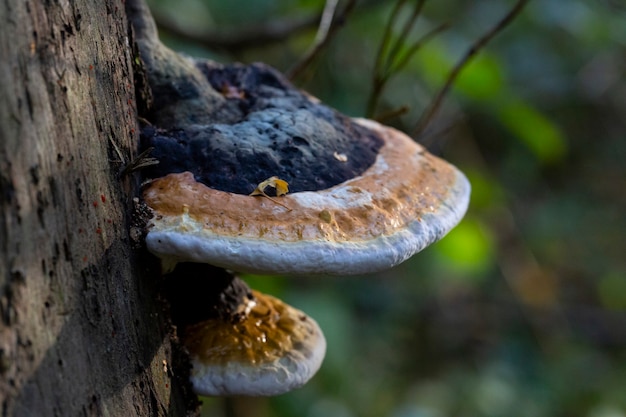This photograph captures an up-close view of a pair of mushrooms growing from the side of a tree trunk in an outdoor setting. The tree's bark, prominently displayed on the left side of the image, serves as the base from which the mushrooms emerge. The top mushroom, significantly larger, has a distinct coloration with a dark blue or blackish center that gradually fades into brown and white, with the edges appearing light blue to white. Below it, a smaller mushroom, partially shielded by the larger one, displays a yellow center with pure white edges. The background is out of focus, creating a blurred backdrop of varying green shades that contrasts with the sharp detail of the mushrooms and tree bark. Additionally, four sticks can be seen protruding in the background, adding to the natural woodland context. The overall lighting of the photograph highlights the textures and colors of the mushrooms, accentuating their intricate patterns and growth.